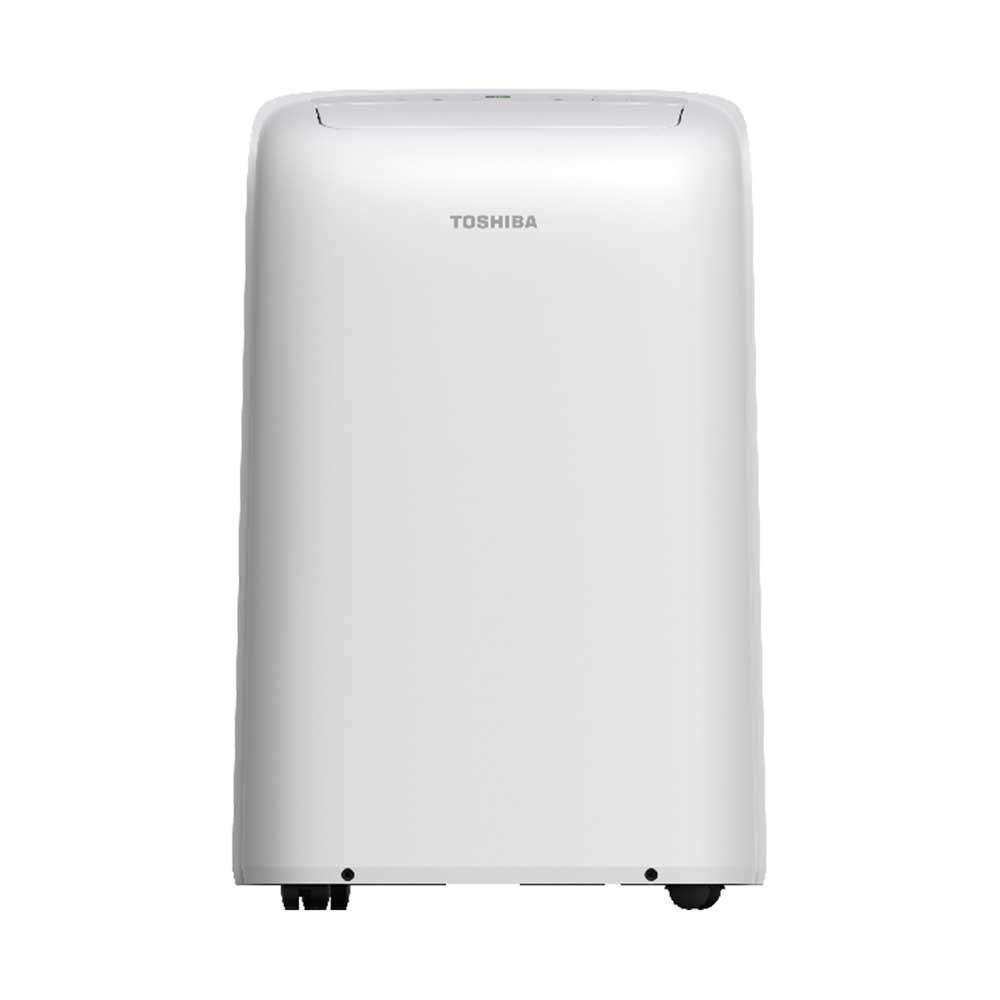This image features a Toshiba-manufactured air purifier with a minimalist design and a solid light gray or white color. The device has a rectangular shape with rounded top corners and is equipped with two small black wheels at the bottom. Just above these wheels are two small black dots or screws. The Toshiba brand name is prominently displayed near the top of the purifier. At the very top, there is a closed flap, likely covering the vents. The background of the image is a plain white, adding to the clean and simple appearance of the machine.